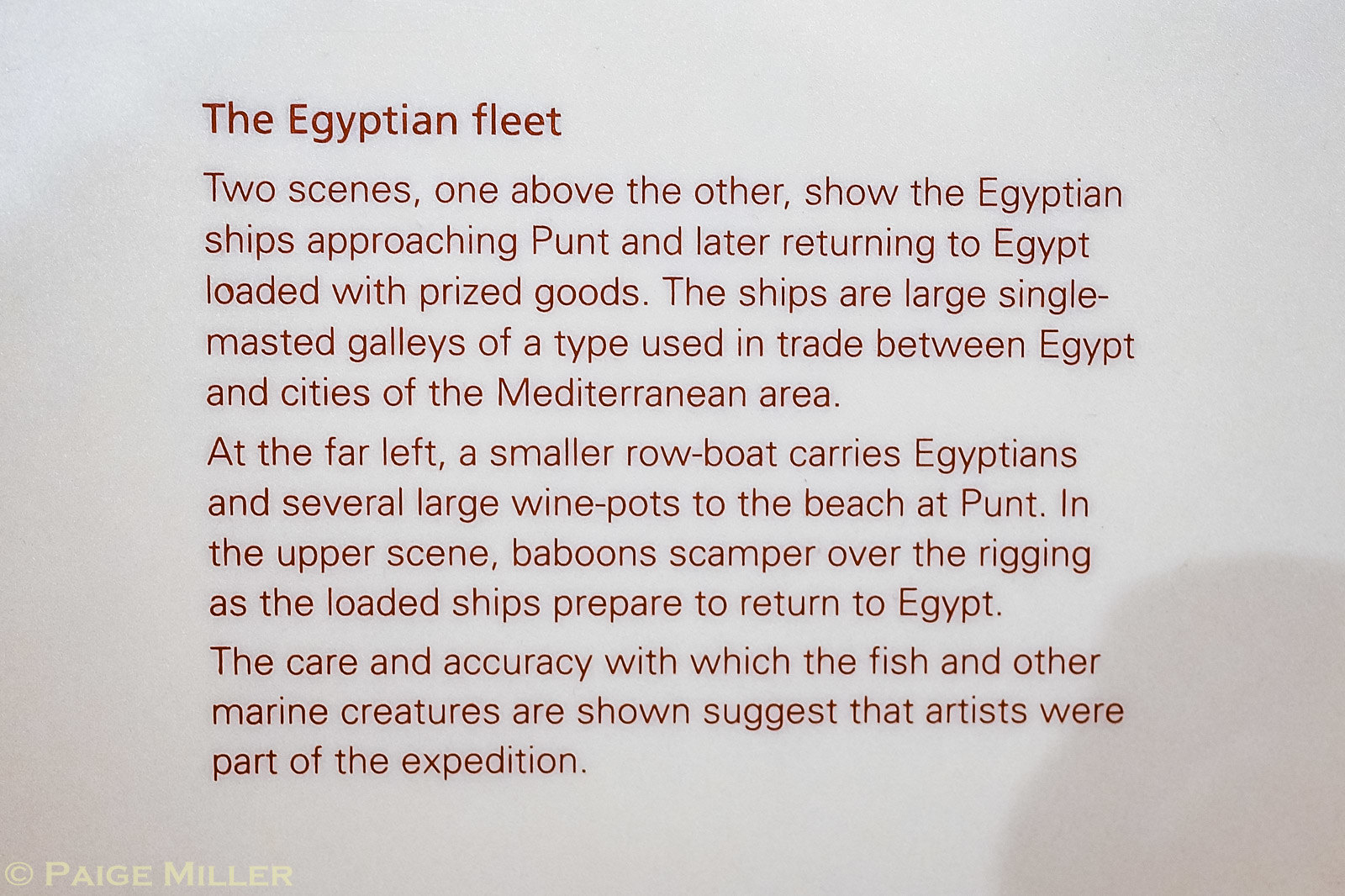This rectangular image, approximately six inches wide and four inches tall, appears to be part of a museum display or an informative slide. It features a gray, shadowed background with red text. The top of the image is prominently titled "The Egyptian Fleet" in bold red lettering. Below this, two detailed paragraphs describe the scenes illustrated.

The first paragraph reads: "Two scenes, one above the other, show Egyptian ships approaching Punt and later returning to Egypt loaded with prized goods. These ships are large, single-masted galleys of a type used in trade between Egypt and the cities of the Mediterranean area. At the far left, a smaller rowboat carries Egyptians and several large wine pots to the beach at Punt. In the upper scene, baboons scamper over the rigging as the loaded ships prepare to return to Egypt."

The second paragraph elaborates on the artistry: "The care and accuracy with which the fish and other marine creatures are shown suggests the artist was part of the expedition."

The lower left corner of the image includes a small copyright symbol (©) followed by the name "Paige Miller" in gold print.